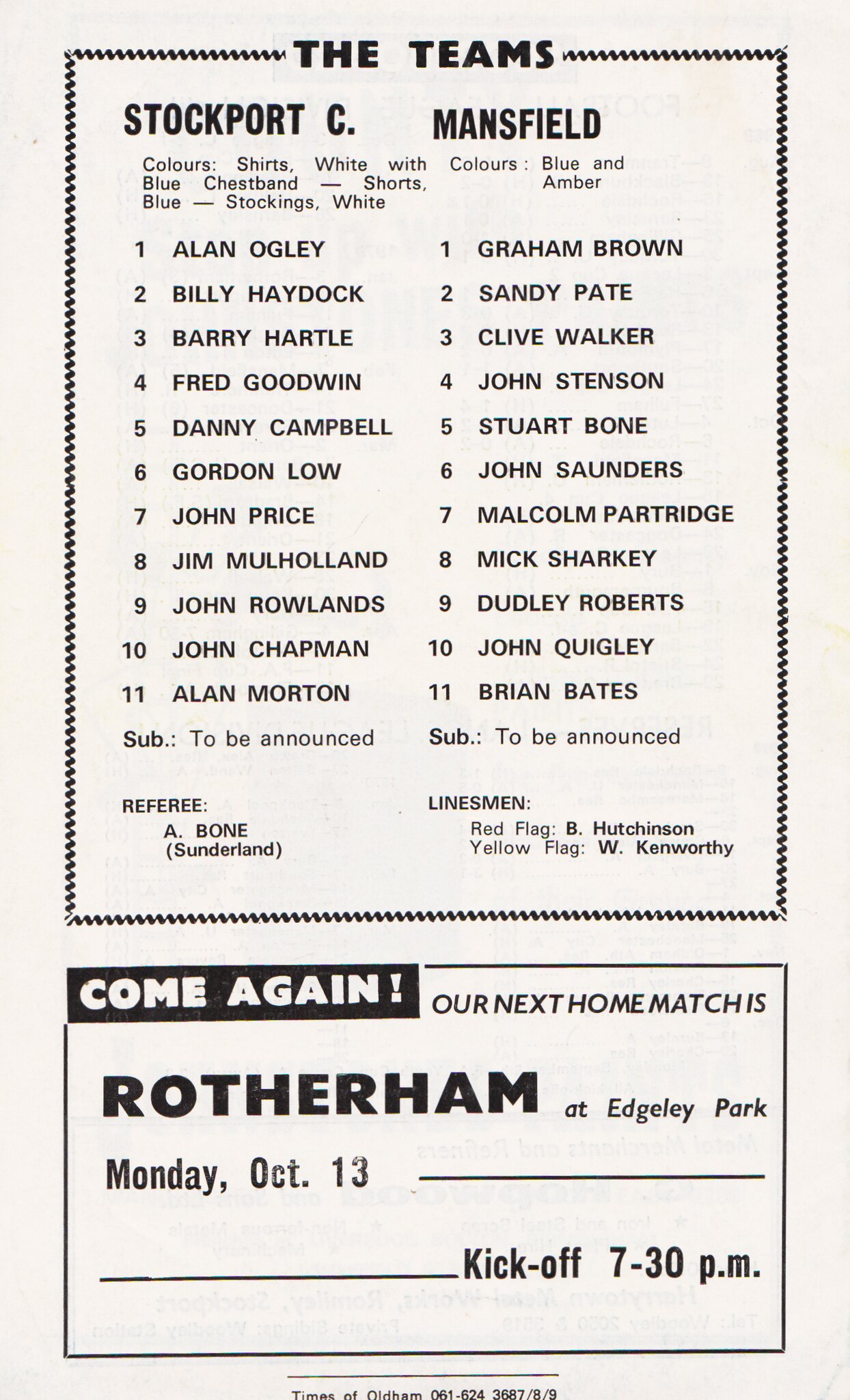The image shows a printed lineup for a match between Stockport C and Mansfield, likely taken from a magazine or program. Stockport C's team colors are specified as white shirts with a blue chest band, blue shorts, and white stockings. The listed players for Stockport C are: 1. Alan Goegli, 2. Billy Haydock, 3. Barry Hurdle, 4. Fred Goodwin, 5. Danny Campbell, 6. Gordon Lowe, 7. John Price, 8. Jim Mulholland, 9. John Rollins, 10. John Chapman, and 11. Alan Morton, with a substitute to be announced. Mansfield's team colors are blue and amber, with their players listed as: Graham Brown, Sandy Pate, Clive Walker, John Stinson, Stuart Bone, John Saunders, Malcolm Partridge, Mick Sharkey, Dudley Roberts, John Quigley, and Brian Bates, also with a substitute to be announced. The referee for the match is A. Bone from Sunderland, with B. Hutchinson (red flag) and W. Kenworthy (yellow flag) as linesmen. Below the team rosters, there's an announcement for the next home match against Rotherham at Edgeley Park, scheduled for Monday, October 13th, with a kickoff time of 7.30 p.m. The document is printed in black type on a cream white background.